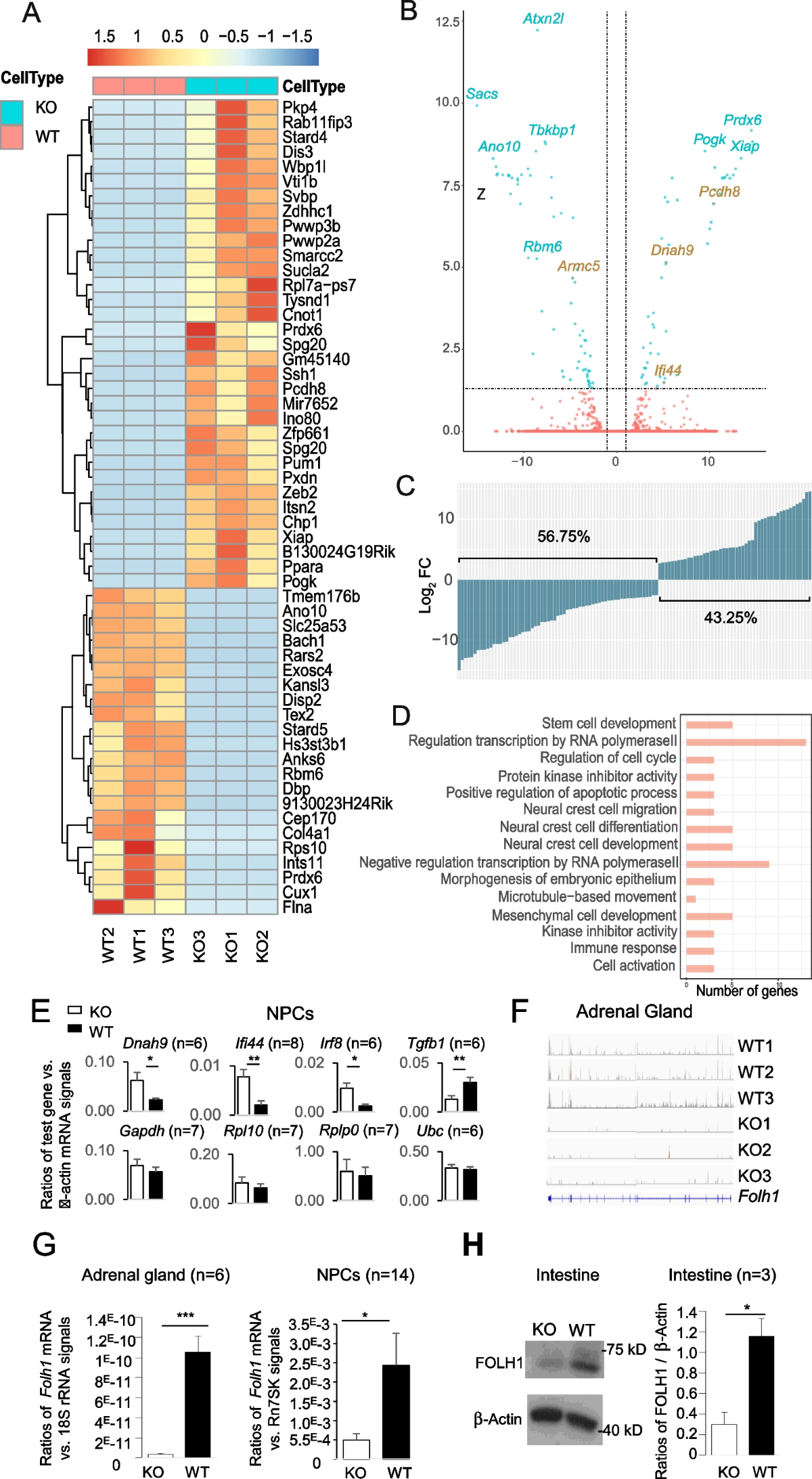The image depicts a complex, detailed layout on a white background showcasing a variety of scientific data visualizations related to cell types. At the top, a scale ranging from 1.5 to -1.5 is displayed alongside a color gradient from red to blue. Below this scale, the main chart is divided into numerous rows and columns filled with rectangular areas illuminated in shades of blue, orange, beige, and light pink. These colors likely correspond to the gradient scale, indicating varying values.

The chart is annotated with labels like WT1, WT2, WT3, KO1, KO2, KO3, and FOLH1, associated with the adrenal gland, and contains headings for sections such as NPC, Intestine, and CELL. It prominently features graphical elements including scatter plots, bar graphs, and dot graphs, each presenting intricate datasets. Labels on the graph indicate cell types marked as KO and WT, alongside notations of specific data points and metrics like 'ratios of test gene versus mRNA signals' and 'Protein Kinase inhibitor Activity'. The image gives a comprehensive, albeit complex, view of scientific information on cells and the body, spanning various types and measurements in a visually dense format.